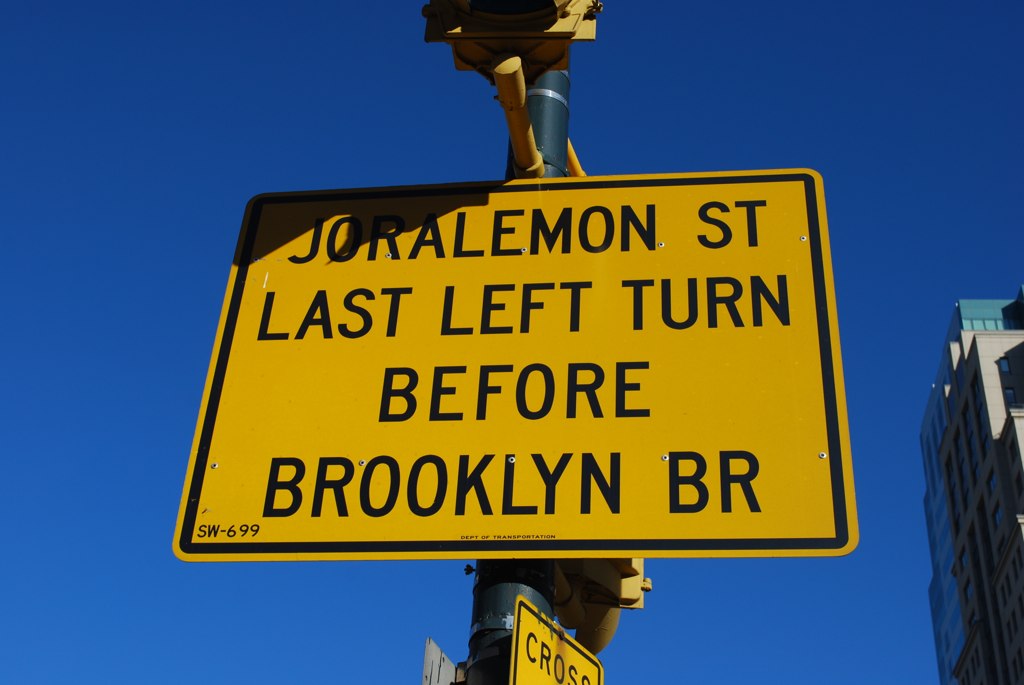This photograph captures a ground-up perspective of a rectangular road sign mounted on a large, dark grey, round metal pole, set against a backdrop of clear blue sky. Above the sign, a street light is visible. The sign itself is a vibrant golden yellow with a black trim, and features the text "Yarlamun Street, last left turn before Brooklyn BR" in bold black ink. To the right of the sign, a tall skyscraper rises, adding an urban architectural element to the scene.